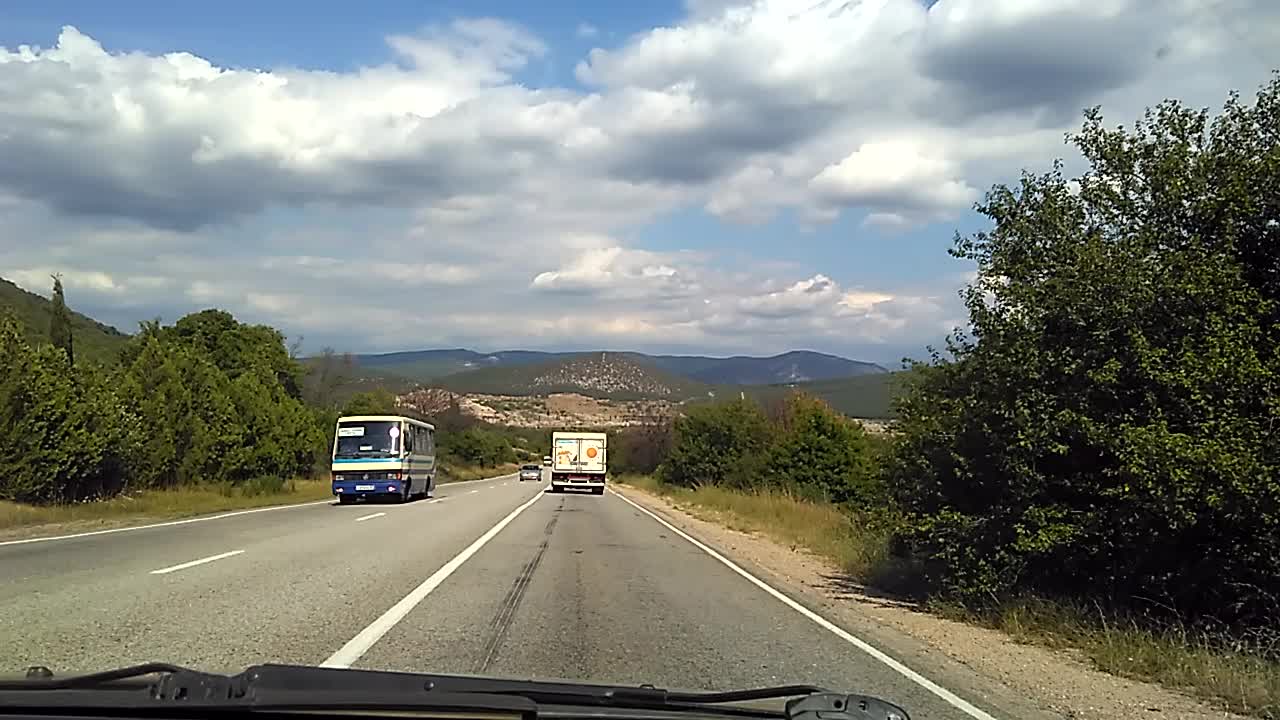This photograph, taken through a vehicle's windshield, captures a scenic roadway scene. In the foreground, a windshield wiper is visible at the bottom of the image. The background is dominated by a sky filled with an array of clouds. Below, majestic mountains stretch across the horizon, creating a dramatic backdrop to the landscape. Flanking the road are lush trees and patches of shrubs and tall grass, adding a touch of greenery to the scene.

The car from which the photo is taken occupies the single right-hand lane, trailing behind a white box truck. On the left, two lanes accommodate traffic heading in the opposite direction. A blue and white bus, with a blue base and white top, travels in the farthest left lane. In the adjacent lane, a small car is driving towards the camera, with another car visible further back. Nestled at the foot of the mountains, a small village peeks through the landscape, completing the picturesque view.